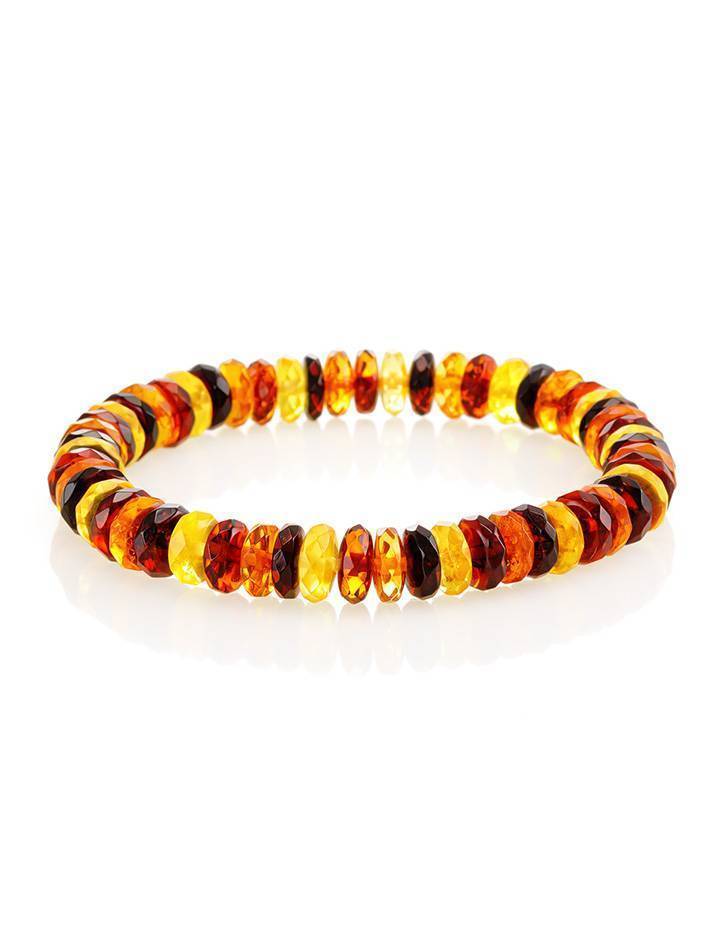The image depicts a detailed bracelet made of assorted beads, which appears to be lying on a plain white background. The bracelet, likely designed to be worn via a stretchy material, features a haphazard yet repeating pattern of different colored beads that resemble small jewels, potentially made of glass or plastic. The beads include opaque and translucent varieties, predominantly in shades of yellow, amber, red, and orange. Notably, the yellow beads stand out as the brightest among them. The colors follow a discernible sequence: a yellow bead, a dark amber bead with some translucence, a reddish bead, and an opaque orange bead, continuing this pattern around the bracelet. The image is taken from an angle slightly above the bracelet, revealing a subtle reflection on the flat, possibly shiny surface beneath, adding a touch of depth to the scene. No person is present in the image, and a small shadow cast by the bracelet is visible, enhancing its three-dimensional appearance.